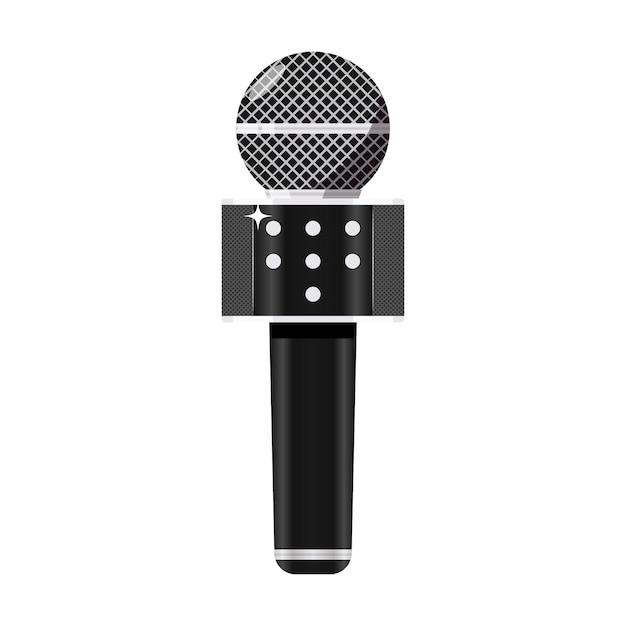This image or drawing, possibly created via computer, depicts a detailed and stylized close-up of a microphone against a plain white background. Starting from the bottom, the microphone features a black circular handle with a prominent silver ring at its base. Moving upward, the next segment includes a wider circular section adorned with a rough-edged design and decorated with an arrangement of seven white dots: three dots in the first row, three in the second, and a single dot in the third row. Just above these dots, on the upper left, there's a small, four-pointed stylized star.

The top of the microphone is a spherical "ball" designed with a crisscross braided pattern, featuring a central silver band akin to an equator line. The sphere appears shaded on one side, suggesting a light source from the left. The entire image is rendered in black and white, with no background elements or identifiable markings, suggesting it is intended for general illustrative purposes.